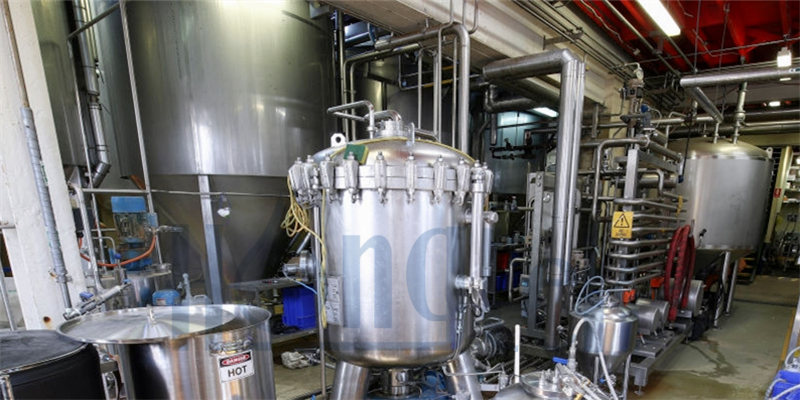The photograph depicts an industrial setting, possibly a brewery or food manufacturing plant, characterized by an array of metallic equipment and fixtures. Central to the image is a large silver machine with a conspicuous green and yellow sponge resting atop it. Surrounding this machine are various pieces of equipment, including numerous silver cylinders connected by hoses, and industrial cookers or large pots, one of which has a prominent "Danger Hot" sign. In the background, an even larger piece of silver metal equipment can be seen, adding to the industrial ambiance. The floor is made of brown concrete, while the ceiling features red lights and red lines that run midway up the walls. The entire scene is dominated by metal pipes and canisters, reinforcing the complex and mechanical nature of the facility.